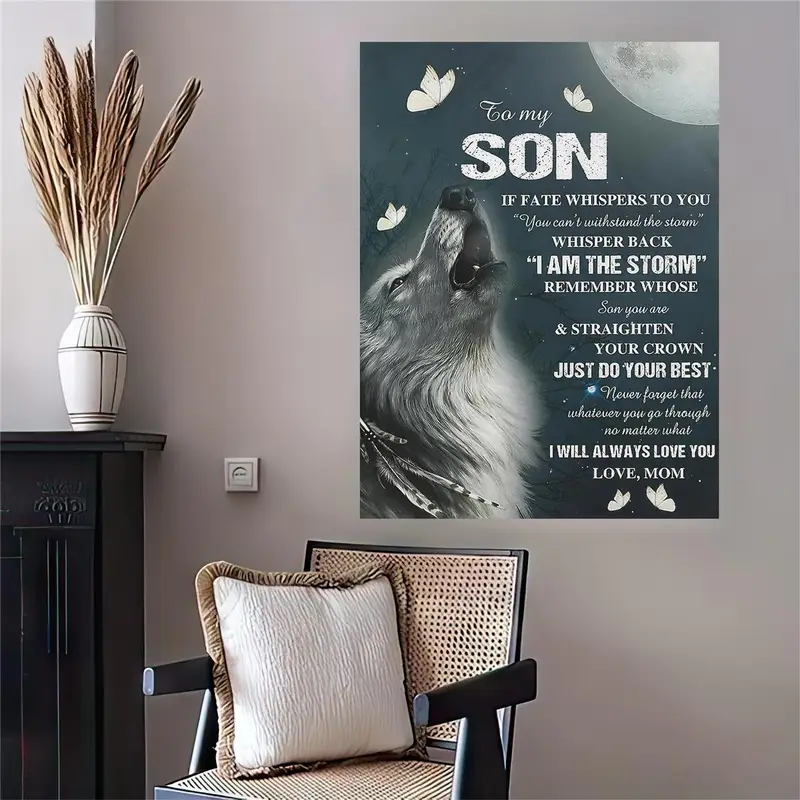In a cozy room setting, a charming wooden table and a small wooden chair with a wicker seat back and cushion are arranged against the wall. The chair features a white and tan pillow at its base. Adjacent to the table is a white vase filled with tufted, brown pampas grass. Above the chair, a large gray and white poster captures attention with its intricate design of a wolf howling at the moon, accompanied by delicate butterflies and feathers in the wolf's fur. The poster's heartfelt message reads: "To my son, if fate whispers to you, you can't withstand the storm, whisper back, I am the storm. Remember whose son you are and straighten your crown. Just do your best. Never forget that whatever you go through, no matter what, I will always love you. Love, Mom." The surrounding ambiance is completed with a European-style outlet on the wall and what appears to be the edge of a fireplace hearth to the left, adding a warm, homey touch to the scene.